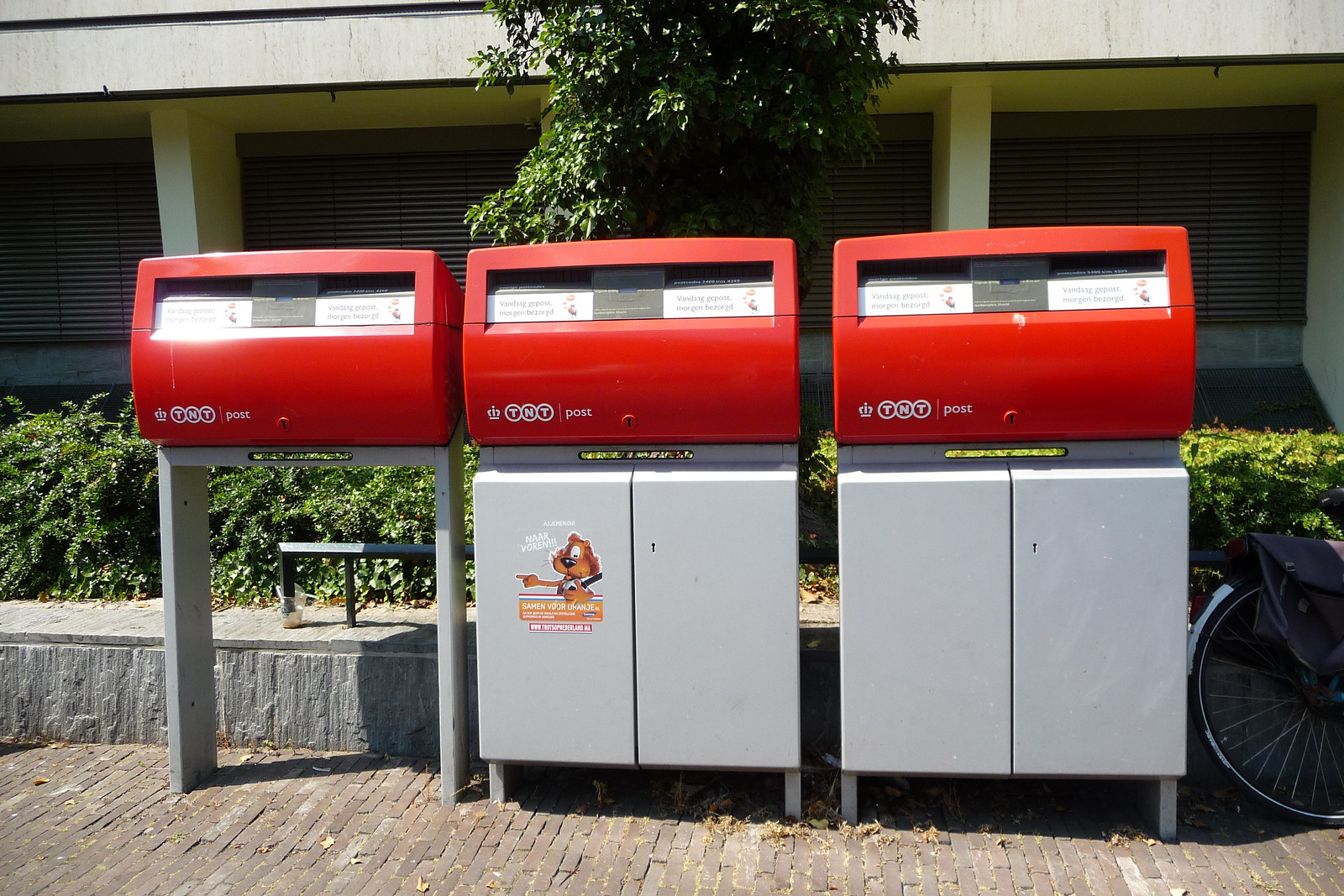This outdoor photograph captures three red-topped postal service machines, standing on a cobbled brick pathway. Each machine features a clear display screen and prominently displays the label "TNT Post" on the top red portion. The two machines on the right have closed grey doors beneath the top section, while the one on the left is missing its doors, leaving an open frame. Notably, the middle machine has a sticker of a cartoon dog on its left-hand grey door. 

The backdrop includes a small wall about a foot and a half high, topped with green shrubbery that runs across the length of the image. Behind the shrub, there's a building with windows that have their shades drawn. Additionally, the rear tire of a bicycle, equipped with a reflector, mudguard, and a black pannier, appears on the right side of the frame, leaning against the concrete pathway.